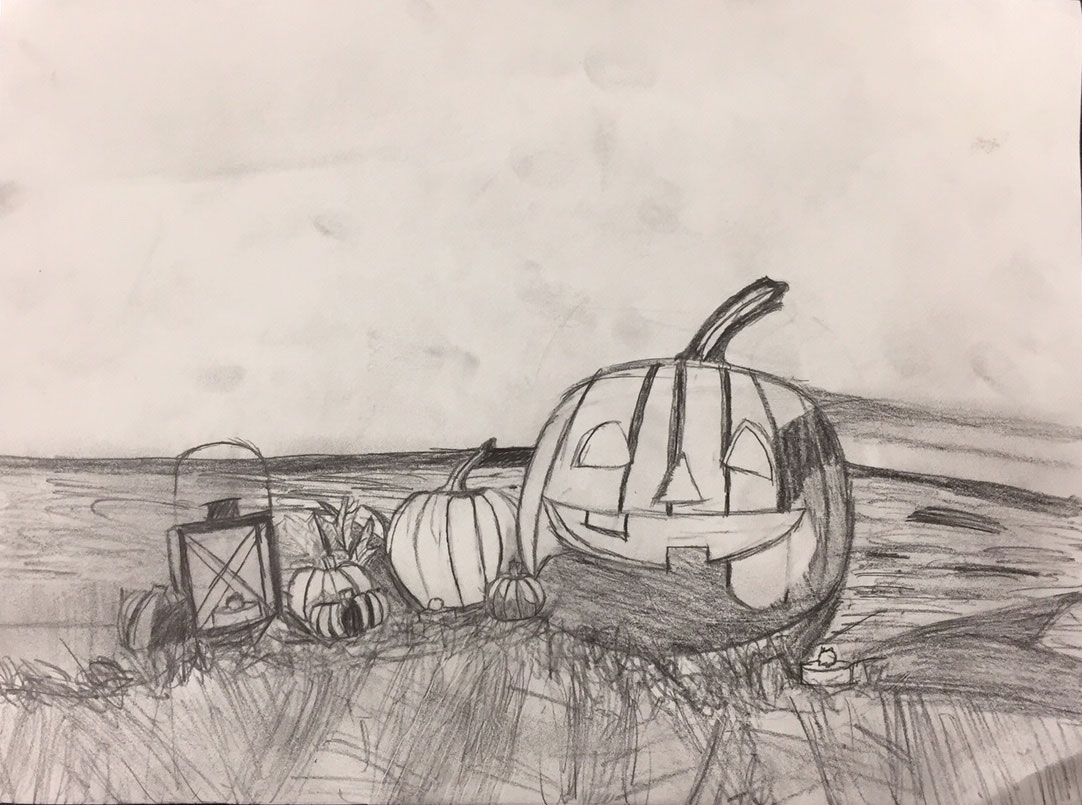This black and white, pencil-drawn image on white paper depicts an autumnal field scene rich with detailed elements. At the left side of the drawing is an old-fashioned lantern with a handle at the top, housing a visible portion of a candle inside. Adjacent to the lantern are a few pumpkins casually scattered on the ground. The central focus of the image is a large jack-o'-lantern with a distinct stem pointing to the right. This jack-o'-lantern features triangular cut-out eyes and a triangular nose, along with a carved mouth showcasing two prominent teeth - one on the top and one on the bottom. The background is subtly implied, keeping attention centered on the charming still life in the foreground. No artist’s signature or any writing is present on the drawing.